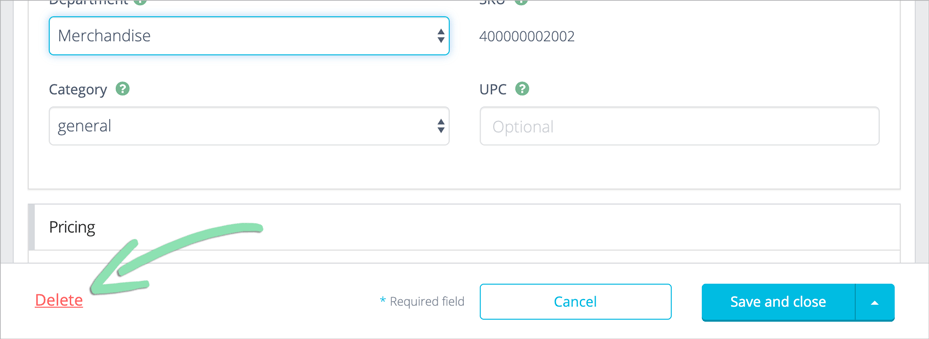Screenshot of a webpage interface, likely part of a merchandise control system. The screenshot is small, and part of the interface is cut off. The visible text includes part of a word suggesting "department." A blue box is highlighted, labeled "Merchandise." Additionally, there's an area marked with "JK" followed by multiple zeros and ending in "2002."

A section is circled in green, displaying "Category?" and indicates "General." Another field, "UPC," is also circled in green and marked as optional. Below these fields, there is a pricing section contained within its own distinct box.

At the bottom of the interface is a prominent red "Delete" button, pointed out by a green arrow originating from the pricing box. This appears to be part of an instructional guide. Notably, none of the fields in this view are marked as required, as indicated by asterisks. 

The footer area features a blue-outlined "Cancel" button with blue text, alongside a blue box with white text labeled "Save and Close." There’s a small arrow icon on this button, suggesting it might open a context menu. The webpage background is a plain white.

Overall, a substantial portion of the webpage is not visible, but the context suggests it belongs to a merchandise management system.